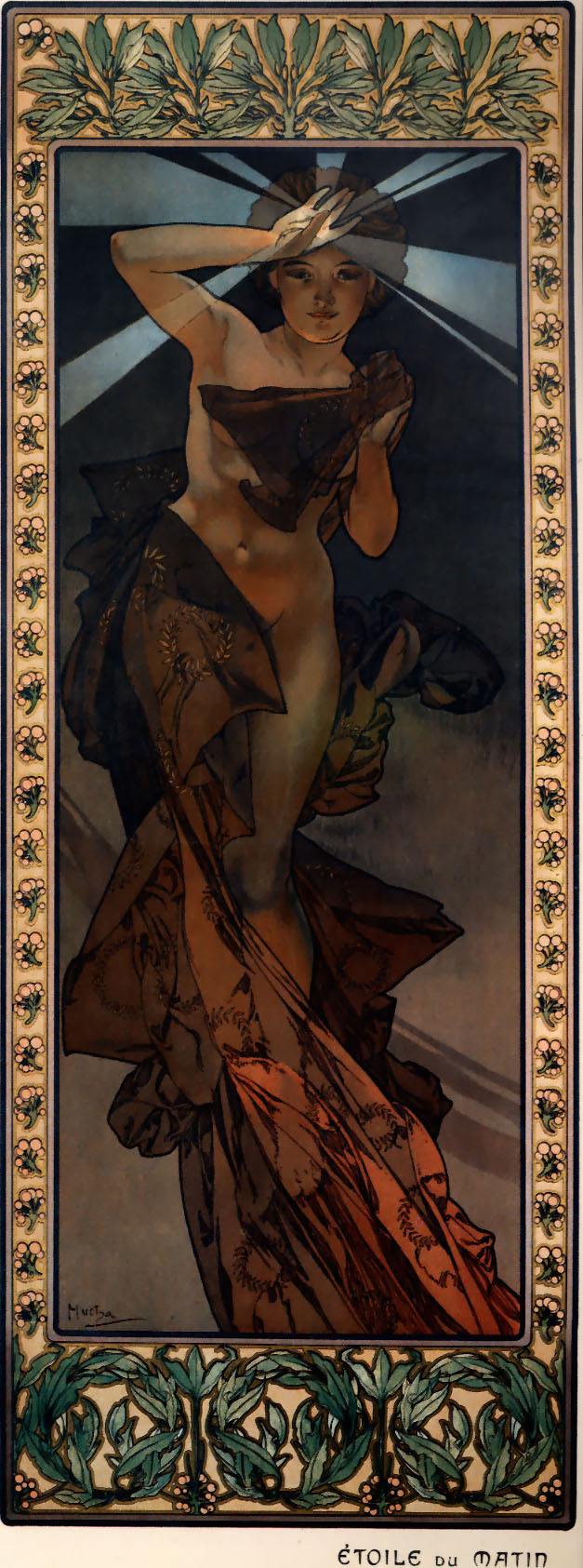The image is an Art Nouveau-style painting, vertically oriented and framed by a cream background adorned with green leaves and floral patterns along the edges. At the center of the composition is a half-naked woman, strategically draped in red robes that cover her legs, hips, and partially wrap around her back to her bust, leaving one breast exposed. Her left arm is raised, with her hand resting dramatically on her forehead, while her right hand grasps the flowing cloth. The woman has short hair, arranged in a halo-like fashion, and light radiates from her head, depicted as rays of varying thickness extending outward in a 270-degree arc. These rays originate from her palm and add an ethereal quality to her appearance, making her seem almost as if she’s floating. The background behind her is dark, enhancing the luminous effect of the light rays. At the bottom right corner, there is text that reads "Atual Du Matin". The overall aesthetic evokes classical Roman elements, which contributes to the painting's timeless, artistic allure.